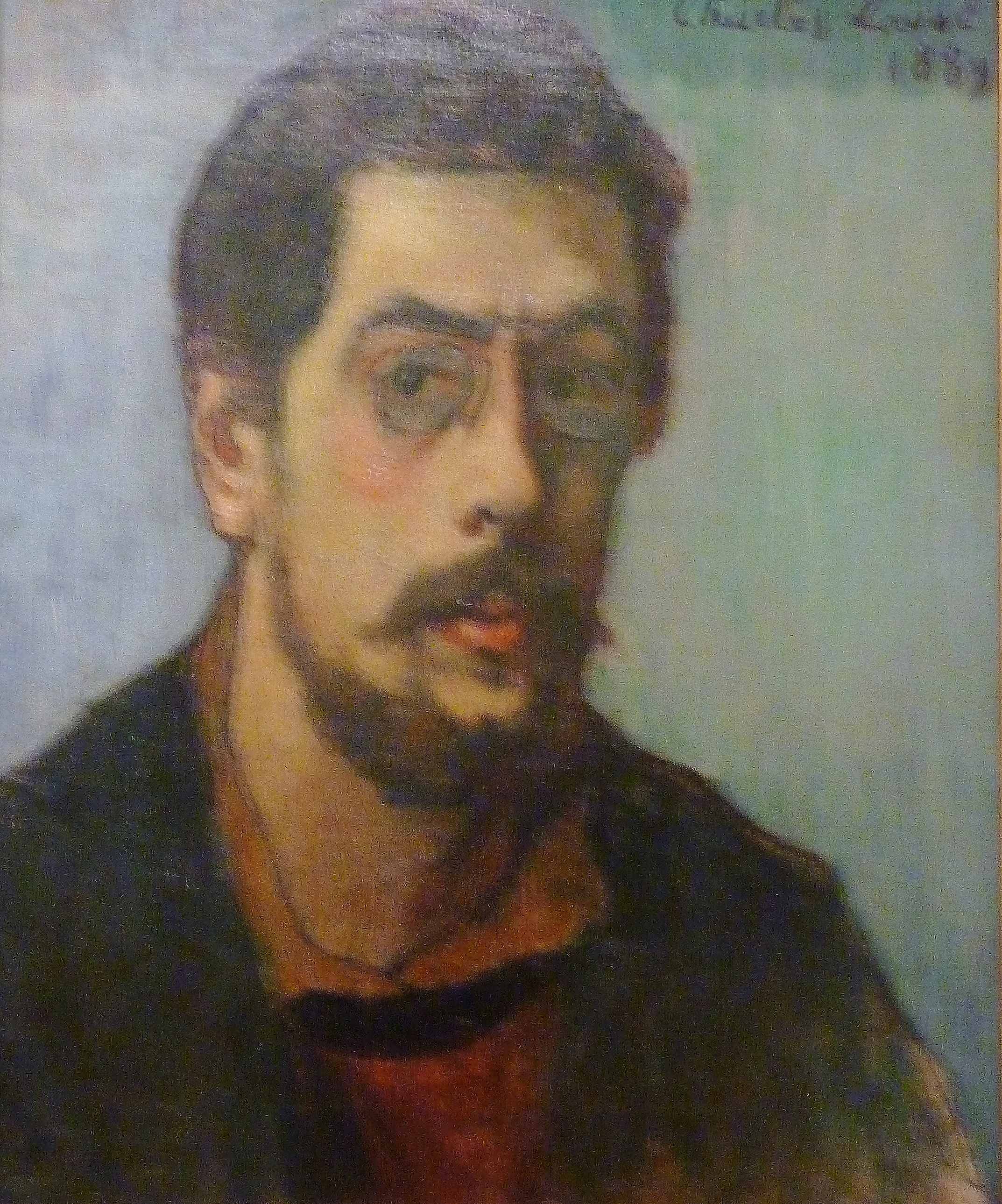This detailed painting, likely a self-portrait created in 1889 by the artist Charles Lever, portrays a serious-looking Caucasian male in his mid to late 30s. He has dark brown hair that partly covers his ears, a matching mustache and beard, and distinct glasses that lack visible earpieces. His striking red lips resonate with the color of his collared orange shirt, which is layered under a brownish-green jacket. The man’s elongated face, capped with an attentive expression, is oriented towards the artist. The background features a blend of aquamarine on the right and a mix of blue and lavender on the left. The artwork appears to be created with oil and pen, with the signature "Charles Lever, 1889" clearly inscribed in the top right corner.